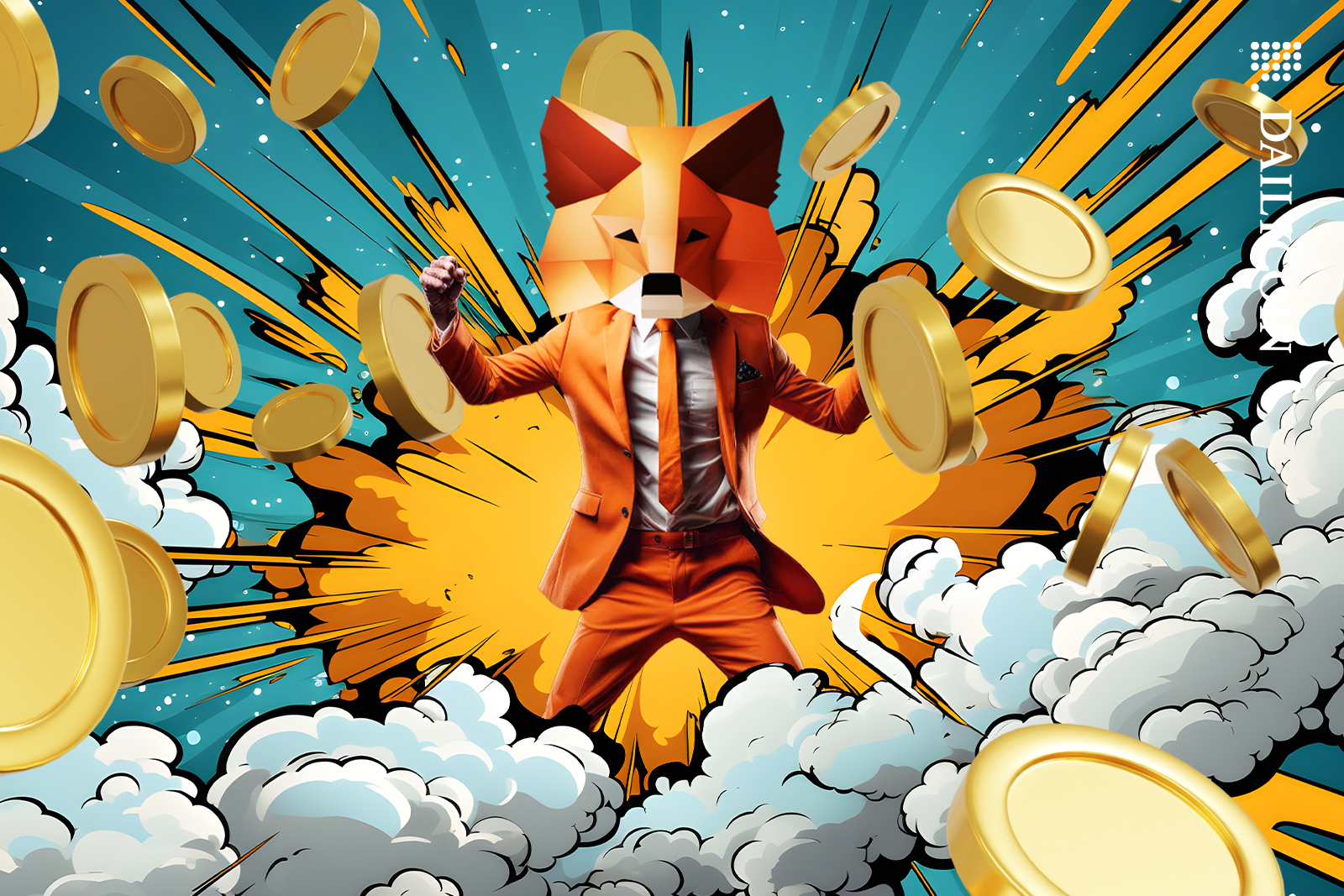The image depicts a vibrant digital artwork featuring a humanoid character with a distinctly 3D, cartoony fox head. The character is dressed in an orange suit with an orange tie over a white collared shirt, and orange trousers. Notably, the fox head is predominantly orange with pointy ears—one orange and one black—and a white mouth. The character strikes a celebratory muscle flex pose in the center of the image.

Behind the fox-headed character, there's a dynamic, comic book-style explosion rendered in yellow and orange hues, dispensing golden coins dramatically. Surrounding the explosion are clouds of white smoke, adding to the scene's exuberance. The background showcases a mix of green and blue with white dots. Additionally, scattered gray smoke clouds can be seen towards the bottom right corner.

In the upper right corner of the image, there is a vertically oriented text logo that reads "Daily Con." This logo adds an extra layer of context to the lively and energetic illustration.